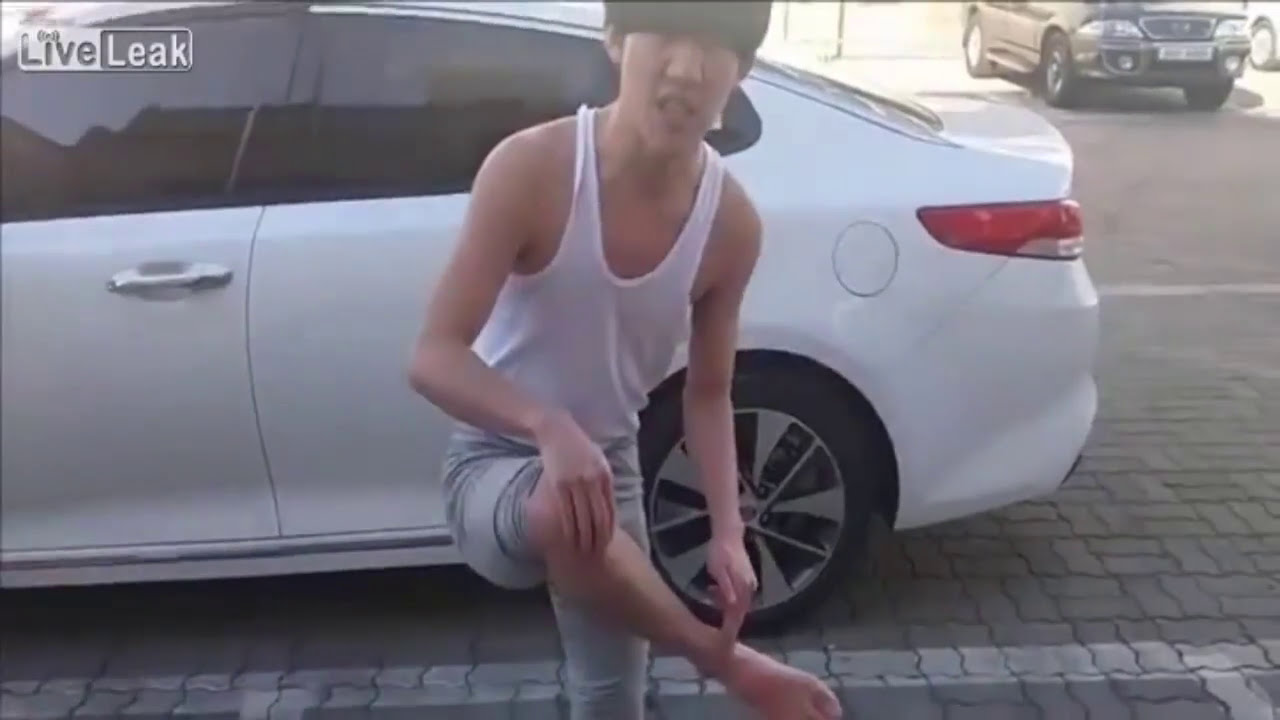An Asian teenage boy stands in a parking lot made of wavy, gray bricks, in front of a white sedan with black accents and a noticeable red taillight. He is wearing a white tank top and grey pants, which are rolled up above his right knee. He maintains a balanced, yet awkward pose, standing on his left leg while pulling his right leg up, with his left fingers touching his ankle and his right hand placed over his bent knee. The boy's gaze is directed upwards towards the camera, though his eyes are obscured, possibly by a bowl cut hairstyle or a hat. The overall image is a bit washed out and slightly blurry, with a 'LiveLeak' logo in the top left corner. To the background, there's another black car parked, adding depth to the parking area marked by white stripes.